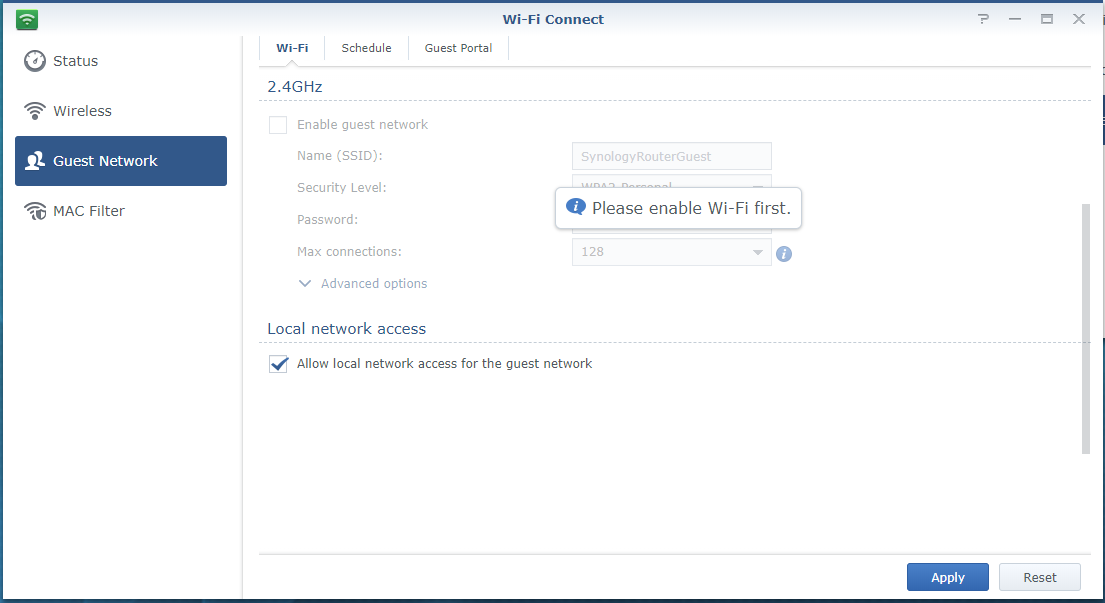The image displays a Wi-Fi Connect screen, although it's unclear whether it's on a tablet or a laptop. The screen has a subtle bluish background. At the top, "Wi-Fi Connect" is written in bluish-gray lettering. 

In the top-left corner, there's a green Wi-Fi icon. In the top-right corner, there are four icons: a gray question mark, a dash, an expand window icon (window within a window), and an X.

The center of the screen features three tabs labeled "Wi-Fi," "Schedule," and "Guest Portal." The "Wi-Fi" tab is selected, indicated by blue highlighting and an indent underneath.

Directly below, "2.4 GHz" is written in blue text with a dashed line underneath it. There's an unchecked checkbox labeled "Enable Guest Network." 

Below this, there are fields for "Name (SSID):", "Security Level:", "Password:", and "Max Connections:". Additionally, there is a bluish-gray down arrow labeled "Advanced Options." The right side displays four greyed-out text boxes with various settings: "Synology," "Router," "Guest," with the fourth box obscured. The bottommost box next to "Max Connections" shows "128" with a little down arrow and a white "i" in a blue circle. Above these text boxes, a dialog box reads "Please Enable Wi-Fi First," with a white "i" in a chat box to the left.

Under the text boxes, the option "Local Network Access" appears with another dashed line beneath it. There's a checked checkbox labeled "Allow Local Network Access for the Guest Network."

On the left side of the screen, a menu lists: "Status" with a clock icon, "Wireless" with a Wi-Fi signal icon, "Guest Network" with two people icons, and "MAC Filter" with a wireless icon and a shield.